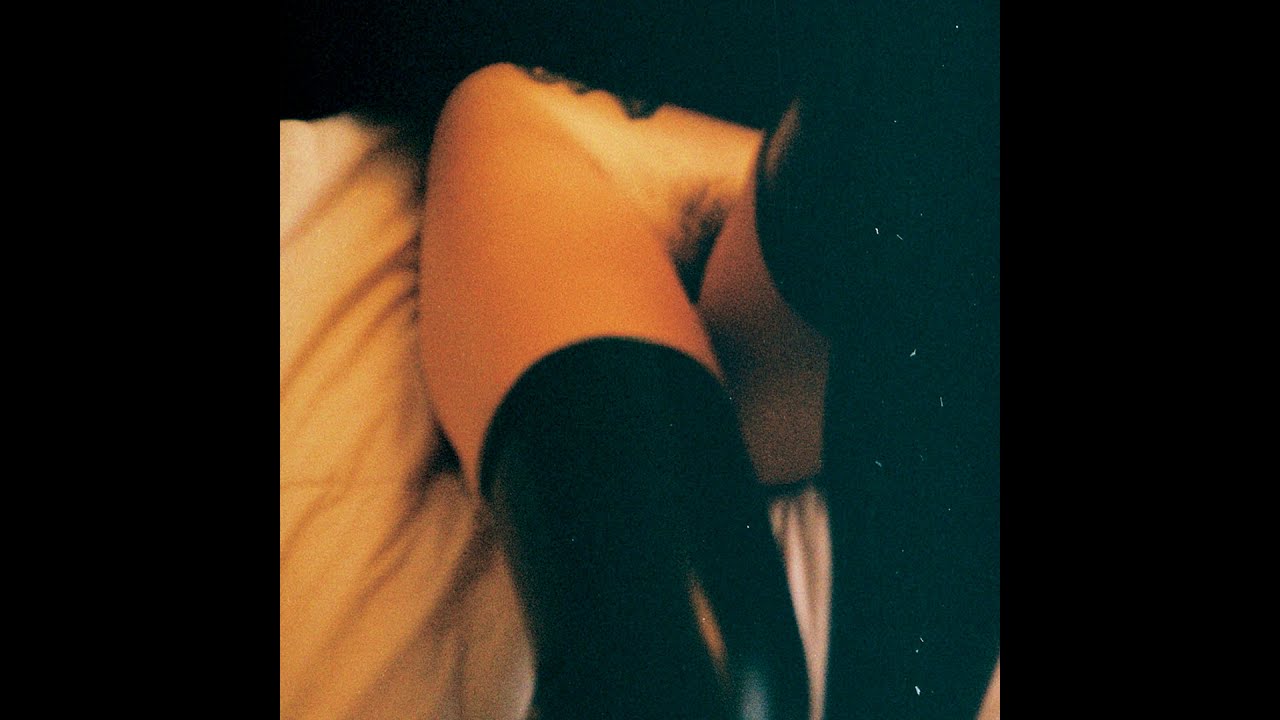This photograph features a bottom-view angle of a woman lying on a wrinkled, off-white or beige sheet, likely a bed. The subject's skin has a light caramel hue and her build appears fairly thin. She is wearing thigh-high, shiny black boots or stockings, made of a material resembling leather or latex. In the image, her left leg is bent at a 90-degree angle, extending upwards, while her right leg is bent and appears to reach downward. The scene includes black bars on the left and right sides of the image. Strands of dark brown hair are visible between her legs, and there's also a mention of a dark, spiky tattoo near the knee area, although this detail is not entirely clear due to the photo's angle and lighting.